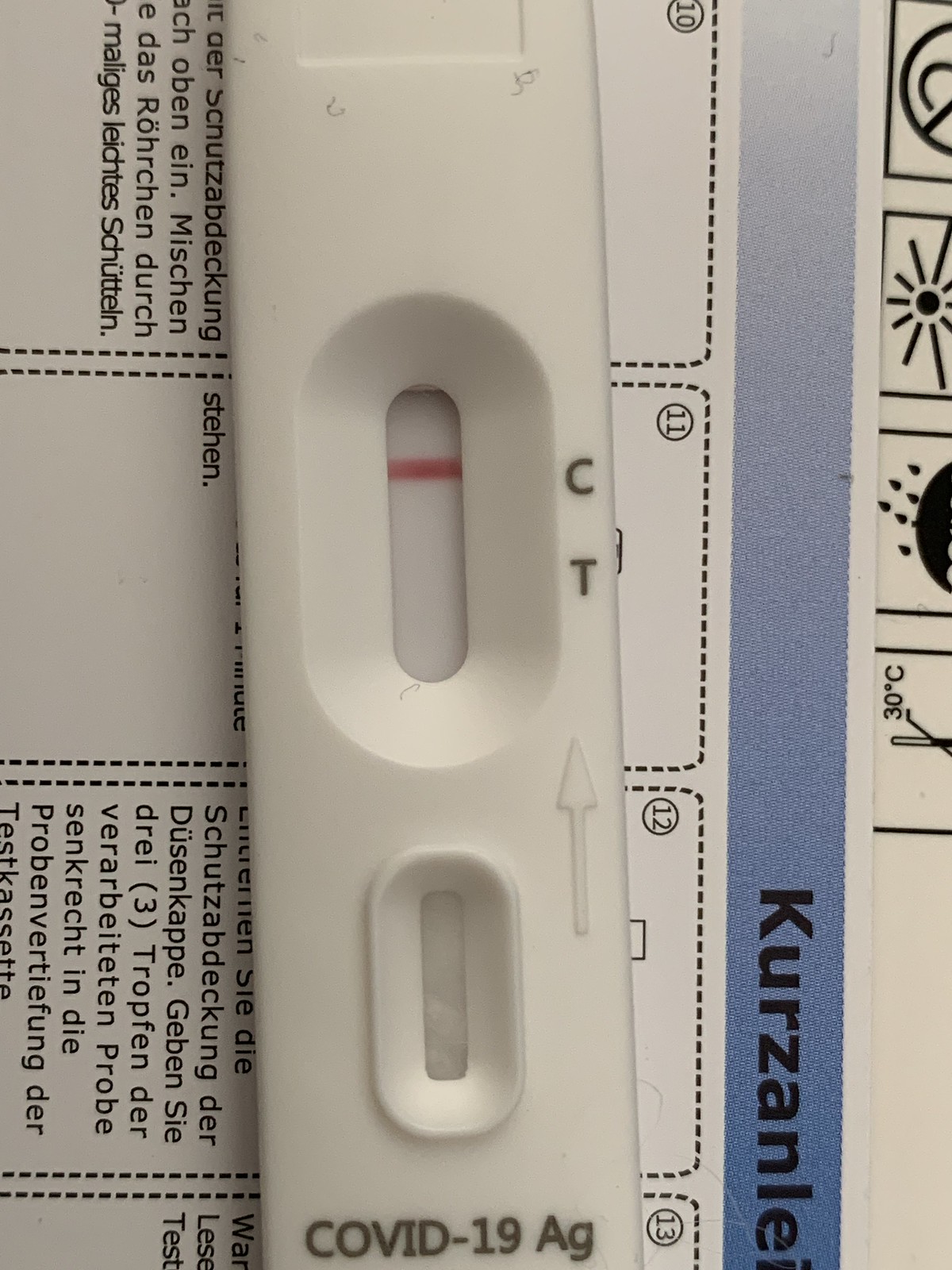A close-up photograph captures a COVID-19 antigen (AG) test placed on a vibrant and colorful surface. The white, rectangular plastic test is positioned vertically. At the bottom in bold black writing, it says "COVID-19 AG." The test features an oval window where a sample liquid is typically dropped. An arrow points upward towards the "C" and "T" indicators on the test, with "C" representing the control line. A distinct red line is visible at the "C" position, confirming the test's validity, while no line is present at the "T" position, indicating a negative result for COVID-19. Underneath the test sits a set of instructions printed on white paper. The instructions, written in German, include various symbols such as black boxes with images depicting 30 degrees Celsius, water, and the sun, which likely refer to testing conditions or guidelines.